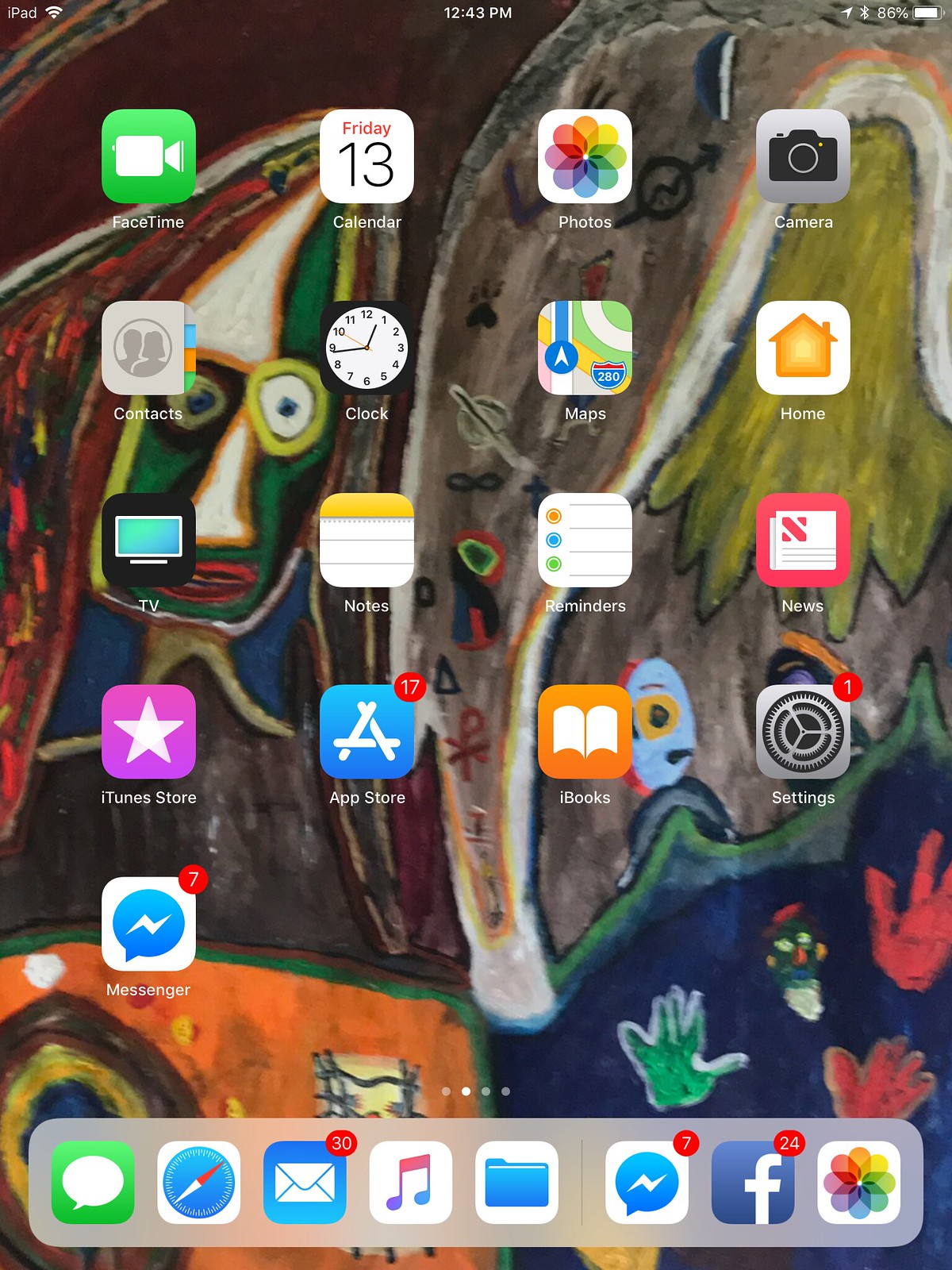The image displays an iPad's home screen with a vibrant and colorful background, featuring an abstract artwork that could either be a child's drawing or a piece of modern art. The iPad is connected to Wi-Fi and shows the time as 12:43 PM with 86% battery remaining. The dock at the bottom of the screen includes frequently used apps such as Mail, which has 30 unread messages, an unidentified app with 7 pending alerts, Facebook with 24 notifications, a music app, Safari, and the Messages app. The main screen is populated with various apps including the App Store (17 notifications), Messenger (7 notifications), Settings (1 notification), Clock, Maps, Home, Camera, Photos, FaceTime, Contacts, TV, Notes, Reminders, News, iTunes Store, and iBooks.